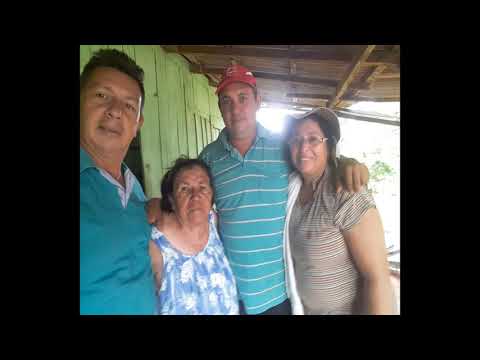In this photograph, we see a closely-knit group of four adults—two men and two women—standing under a wooden awning or canopy, seemingly on a covered porch or patio. Bright sunlight frames the group from behind, highlighting their warm expressions and comfortable posture. 

Starting from the left, the first person is a man in his mid-40s wearing a blue polo shirt with a white-stitched button area and two unbuttoned buttons at the collar. He has brown hair and is slightly smiling, his body angled toward the right while he looks directly at the camera. Beside him stands an older woman, possibly in her 60s or 70s, dressed in a sleeveless blue and white blouse. She is shorter and faces the camera with her body also angled to the right.

Next to her is a taller man, also appearing to be in his 40s. He is wearing a blue and white striped polo shirt with the collar unbuttoned, accented by a red baseball cap on his head. His facial expression is neutral, but he stands in a relaxed posture, possibly with his arm around the woman to his right, indicating a close relationship. This woman is dressed in a blouse with blue and red stripes and wears glasses and a tan hat. She appears to be in her 50s or 60s and is smiling warmly at the camera.

The group seems intimately connected, perhaps family members, with their positioning and body language suggesting a bond of togetherness against the backdrop of sunny weather and greenery.